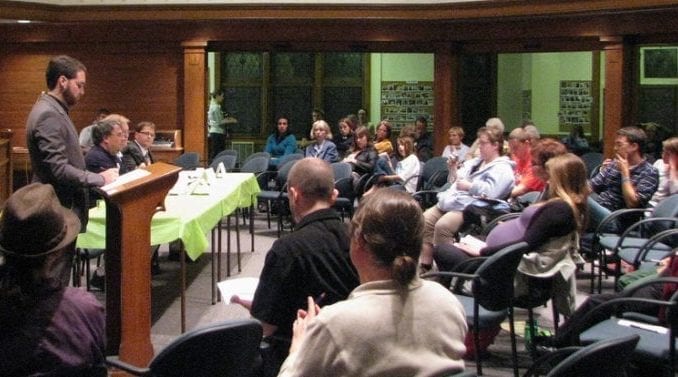The image depicts a meeting, likely at a City Hall or town hall, set inside a spacious room with large windows and wooden columns. At the center of attention is a man in a suit with short brown hair, who is speaking at a podium and reading from a paper. To his left, a table covered in a green cloth hosts three other men who are listening attentively. The audience, consisting of about 20 to 30 men and women of various ages—including a pregnant woman and an older man wearing a hat—are seated on black plastic and metal chairs arranged in rows. A gray floor underlies the scene, and through the windows, a person can be seen walking in the hallway outside.